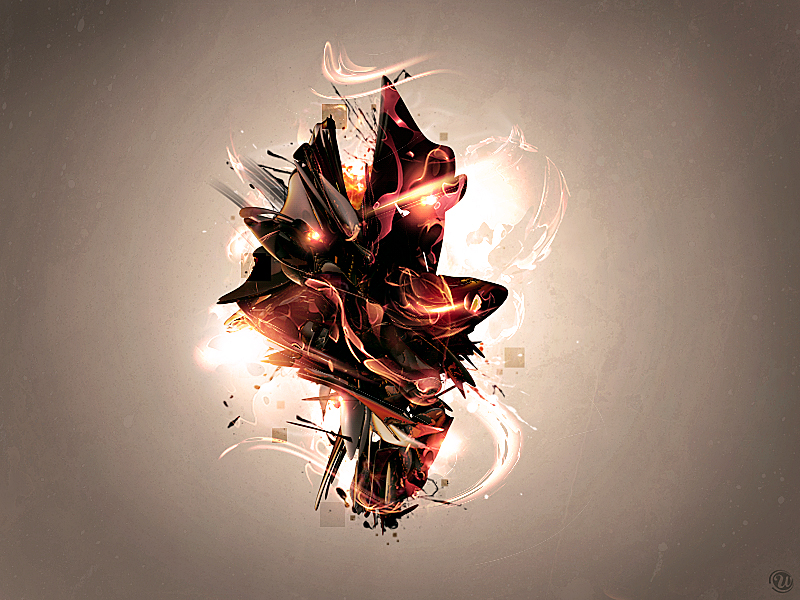The image appears to be an AI-generated illustration characterized by a surreal and abstract design. Dominated by a central, enigmatic, possibly magical object, the image features metallic elements that seem to burst from the center. This main subject has a complex interplay of colors, primarily red and black, with reflections and highlights that create areas appearing orange, especially where hit by an intense, glowing white light. Surrounding this focal point, the background is a mix of pale and dark brown hues with splashes of beige, giving it an earthy texture. The overall composition is suggestive of a high-contrast scene, with a spotlight effect on the metallic object. Notably absent is any written text. In the bottom right corner, there is a logo resembling a "U," while a watermark on the bottom left bears a resemblance to the WordPress logo.